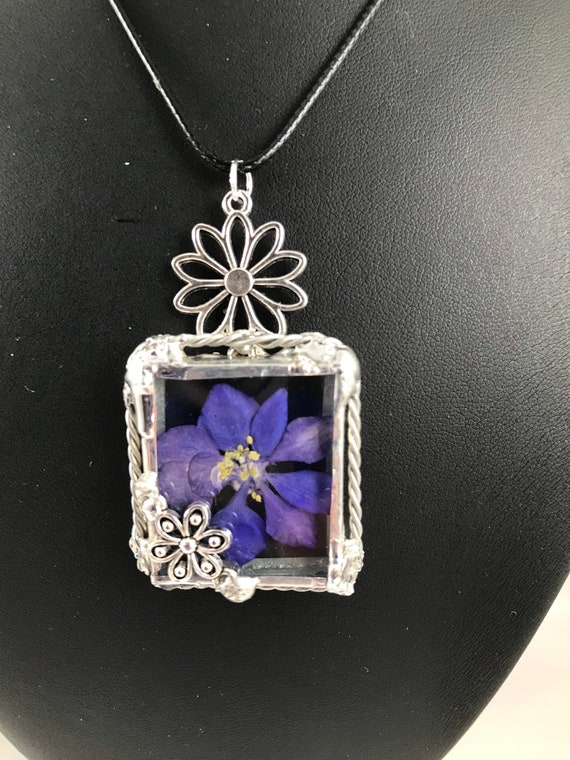This is a color photograph of a necklace displayed against a faux black leather backdrop that mimics the appearance of a human neck and chest. The necklace features a striking pendant hanging from a black cord. The pendant itself is a complex creation, with a stylized daisy-like silver flower at the top, complete with intricate filigree designs. Suspended from this flower is a square pendant framed in elaborately worked, albeit unattractive, silver metal that encases a delicate blue and purple flower. This flower, featuring a yellow center with stamens, has been carefully preserved and flattened between either two plates of glass or transparent epoxy. The pendant exhibits both the craftsmanship involved in its creation and the preserved beauty of the tiny flower within. The image is set against a black background that subtly fades to gray in the upper right corner, enhancing the focus on the detailed craftsmanship of the necklace.